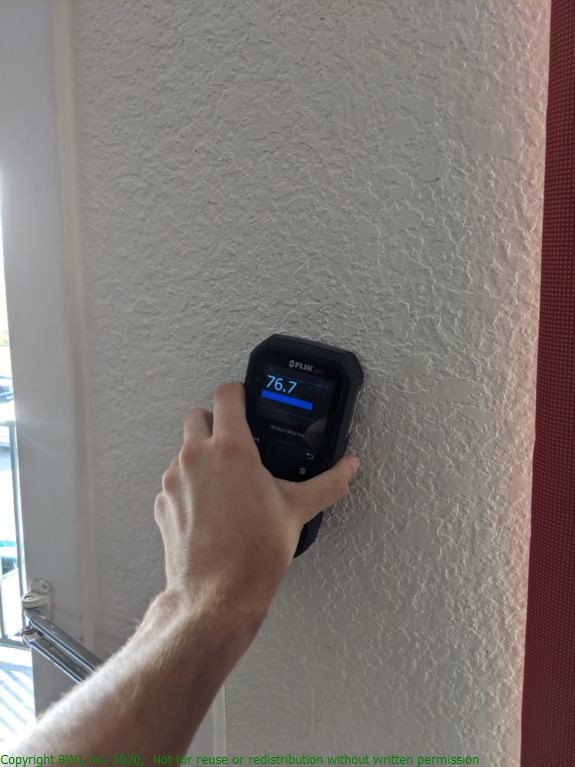A white individual is holding a black electronic device, likely a stud finder, against a textured white wall with their left hand. The device has a digital display showing a reading of 76.7 in white digits, accompanied by a blue line beneath the numbers and some unreadable white text, presumably the brand name, above the readout. Below the device and towards what seems to be the bottom of the image, there are additional components visible, such as pipes and a hinge, suggesting the setting might be near a tall freezer or refrigerator. On the left side of this appliance, there appears to be a silver knob or handle typically used for opening a freezer door. On the right side of the image, an abstract red patterned element, possibly a wall or a piece of fabric, disrupts the predominantly white and metallic aesthetic.